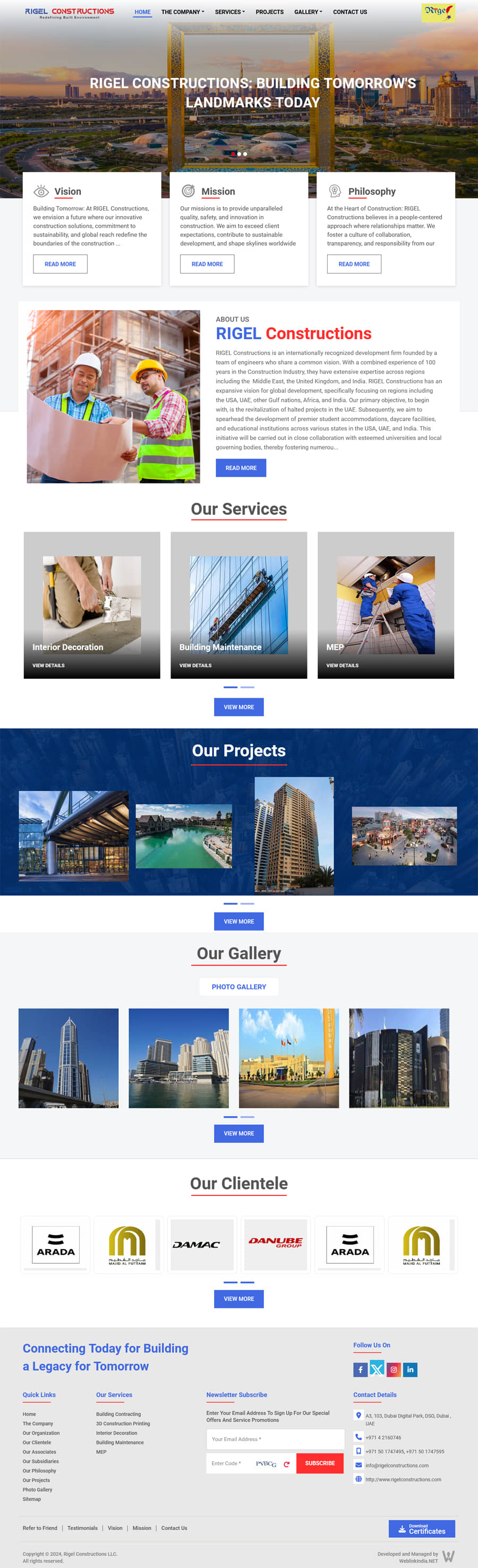This image showcases the homepage of Rigel Constructions' website. The top navigation bar features several tabs: Home, Company, Services, Projects, Gallery, and Contact Us. Notably, the Company, Services, and Gallery tabs have dropdown menus, indicated by small upside-down triangles, which reveal additional options upon hovering.

Dominating the central portion of the page is a striking cityscape framed in yellow. Superimposed on this frame are the prominent words "Rigel Constructions: Building Tomorrow's Landmarks Today," capturing the essence of the company's mission.

Directly below the navigation bar, the page introduces three core philosophies of Rigel Constructions, each housed in separate, easily distinguishable boxes. Following this, the "About Us" section provides a comprehensive overview of the company’s ethos and background.

Sequentially cascading down the page are well-organized sections dedicated to their services, projects, gallery, and clientele. Each section is represented with distinct boxes, housing three to four photographs of various buildings, showcasing the range and quality of Rigel Constructions' work. This detailed layout ensures clear and easy navigation, offering a visually compelling insight into the company's capabilities and achievements.